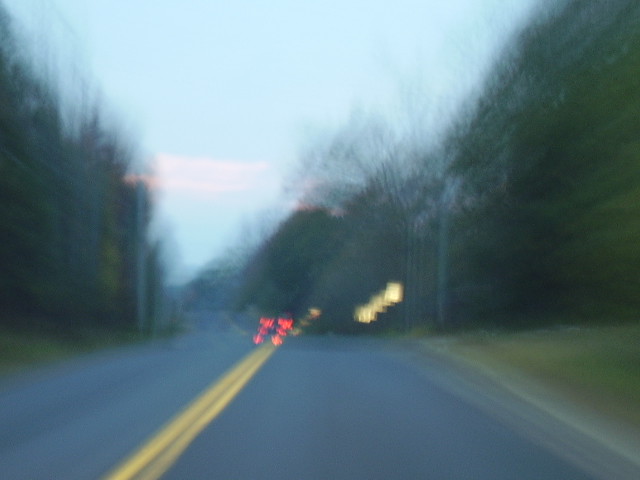A blurred image captured from a car’s windshield, likely taken from a moving vehicle such as a police car or another camera-equipped automobile. The motion blur affects the entire scene, blurring the trees which line both sides of the highway and giving a sense of speed. Faint lights on the left and a string of white light towards the middle add abstract elements to the scene. Grass is visible along the road edges, which is divided by a double yellow line, indicating a no-passing zone. Ahead, a car’s twin tail lights shine brightly in the blurry image. The road appears straight initially but seems to curve to the right further ahead. Clear blue skies with minimal clouds provide a contrasting backdrop to the dynamic, blurred foreground. There are also minor reflections visible on the windshield, adding depth to the overall composition.